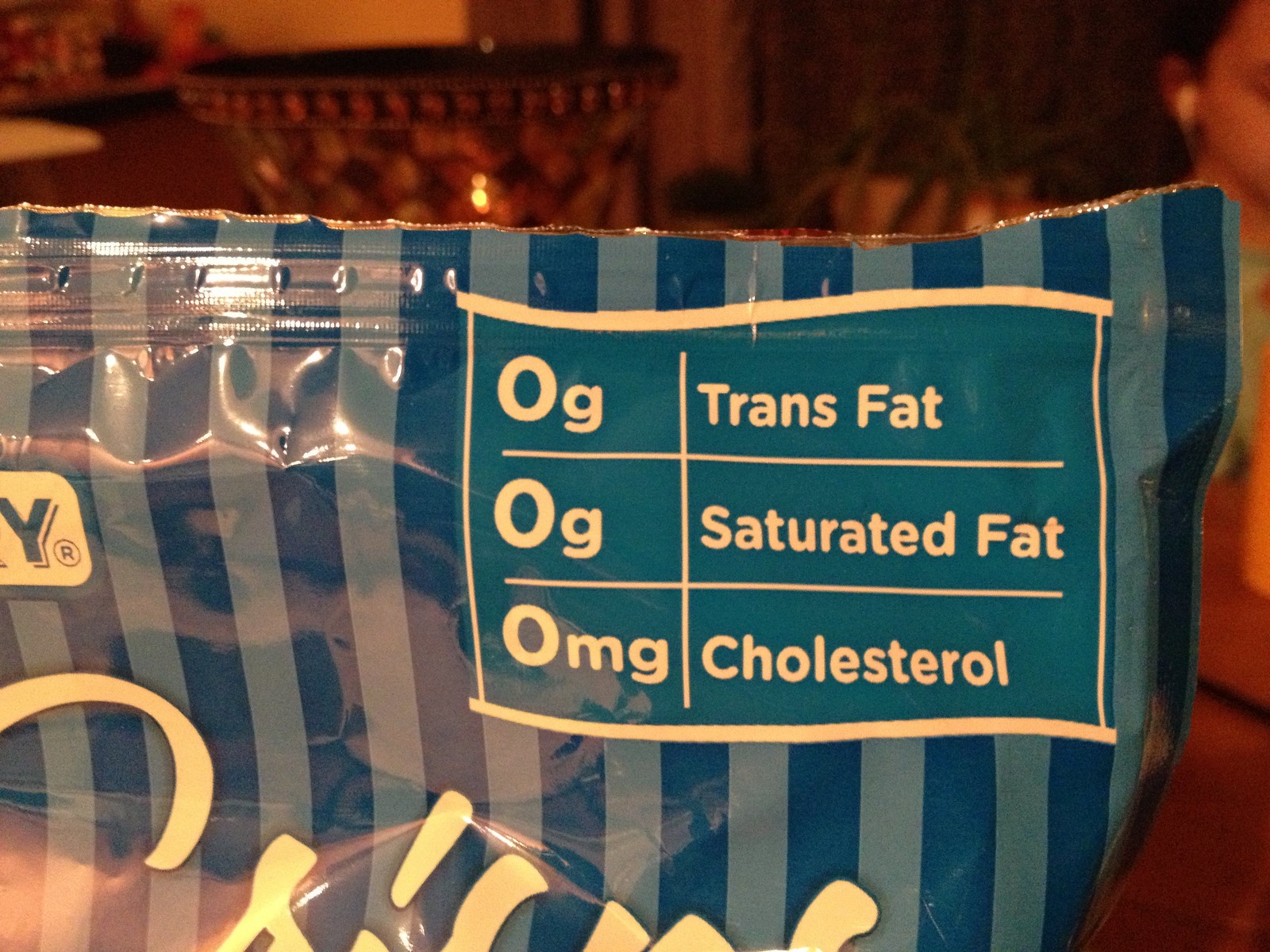In this photo, a partially opened plastic bag of snack foods is prominently featured. The bag is designed with a convenient resealable top, ensuring freshness. The packaging is decorated with alternating light blue and dark blue stripes, particularly noticeable in the right corner. Within a small box on the bag, health information is proudly displayed, stating "zero grams trans fat, zero grams saturated fat, and zero milligrams of cholesterol" in white text. In the background, a woman is standing to the right, wearing either earrings or ear pods. Above the bag, various items are visible, including a lamp, a candle, or possibly a pot, adding to the domestic ambiance of the scene.